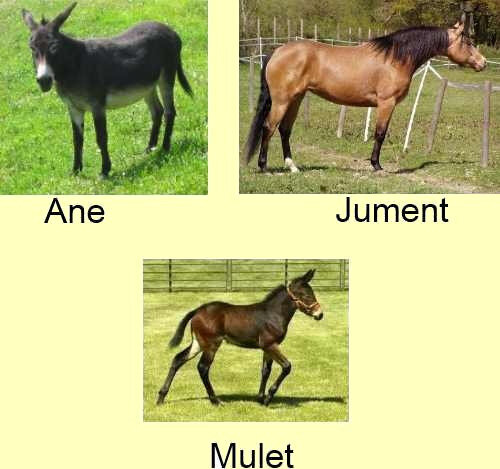The image consists of three distinct animal portraits arranged in an upside-down triangle style: two images on top and one centered below. The top left picture showcases a reddish-brown mule standing on short green grass. The mule, looking directly at the camera, has the text "A-N-E" below it. To the right, another image features a brown horse with a black mane and tail, standing beside a dilapidated wooden fence on a grayish field. The horse, which has one white foot and is gazing to the side with its head over the fence, has the caption "J-U-M-E-N-T" underneath. The bottom center photo portrays a dark brown mulet (a mule-like animal), positioned on a green field with a steel gate in the background. This animal, appearing to prance and looking to the right, is labeled "M-U-L-E-T". The background of all three images is a light yellow shade.